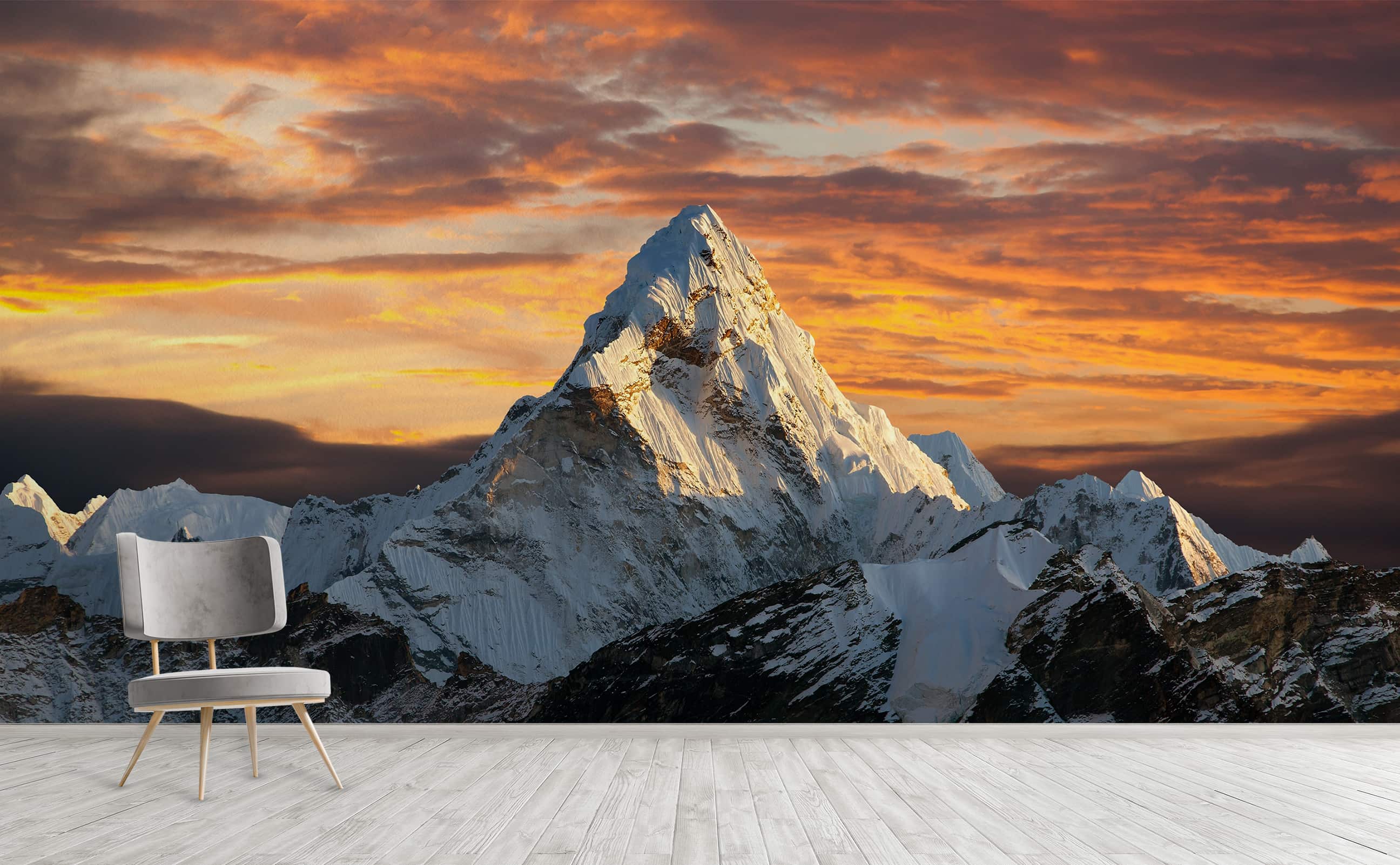The photograph captures a striking mountain scene at either sunrise or sunset, characterized by an array of golds, oranges, reds, purples, and dark clouds that streak across the sky. Dominating the center of the image is a tall, stark white mountaintop, accompanied by slightly smaller, snow-capped peaks displaying dark, shadowy areas. In the foreground, a modern chair with a curved back, flat pancake-like seat pad, and blonde wooden legs sits on a white wooden deck, turned away from the majestic mountain scenery. This captivating and detailed image offers a blend of natural beauty and contemporary design elements.